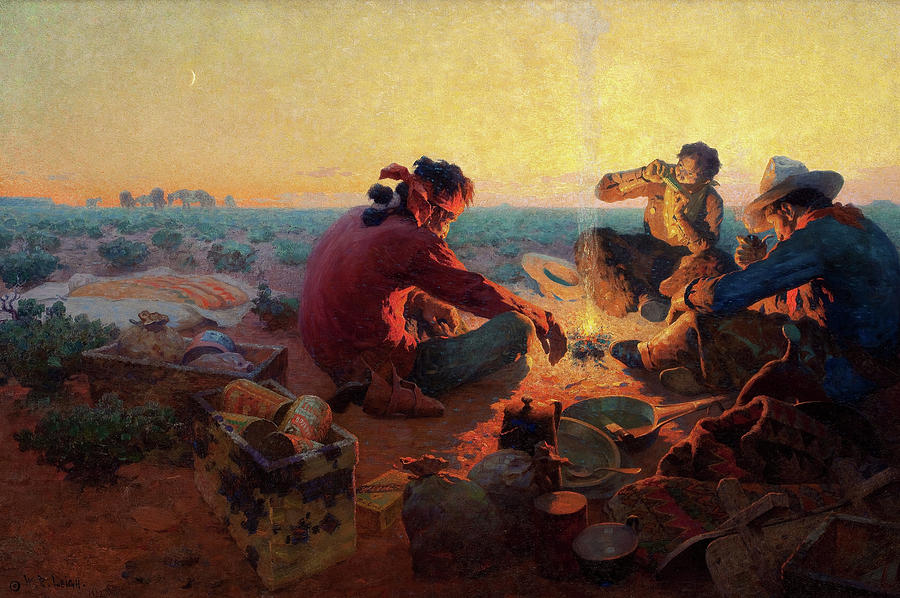This detailed scene captures a nostalgic, old-time oil painting depicting three cowboys gathered around a campfire in a desolate desert landscape during the sunset, with a sky aglow in vibrant shades of orange and yellow, and a sliver of the moon emerging in the distance. The cowboys are surrounded by sparse, low-lying shrubs, and we spot here and there animals in the background, which, though indistinct, appear to be horses or cows. 

The central figure, adorned in fur chaps and a neckerchief, sits playing a harmonica, with his hat placed beside him near a sleeping pallet. To the right, another cowboy, donning leather chaps and a cowboy hat, smokes a pipe and is positioned near his horse's pack. The third figure is distinctive with a red shirt, jeans, a red fabric tied around their forehead, and long hair. This person has a gun holstered at their waist and appears to be thoughtfully tending to the fire, absentmindedly staring into the flame.

Scattered around them are utilitarian items, hinting at the rustic meal they've just shared: metal dishes, silverware, pots and pans, all complemented by the presence of boxes filled with supplies like canned goods, flour, and canteens. A tea kettle adds a homely touch to this rugged outdoor tableau, illustrating a moment of camaraderie and routine in the stark beauty of the plains.